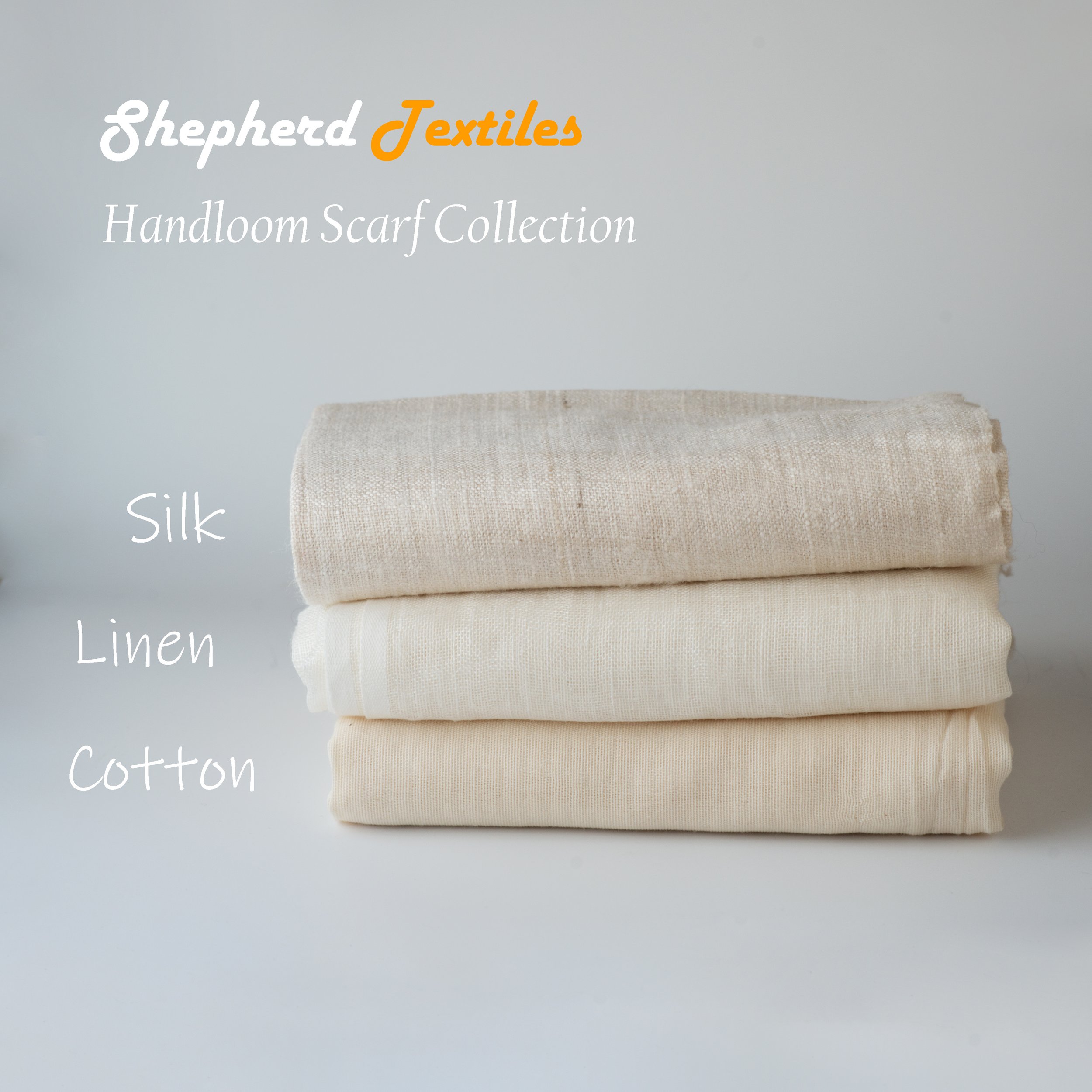The image depicts an advertisement for Shepherd Textiles' Hand Loom Scarf Collection against a light gray background. At the top, "shepherd" is written in white, followed by "textiles" in orange. Beneath that, in white letters, it states "hand loom scarf collection." Centrally positioned in the image is a neatly stacked pile of three scarves, each labeled with its respective material. The top scarf, labeled "silk," has a darker beige hue. The middle scarf, marked "linen," is a more pristine white. The bottom scarf, tagged "cotton," exhibits a creamy color. All scarves fall within a natural beige color range, with subtle differences in shading and texture that are clearly discernible.